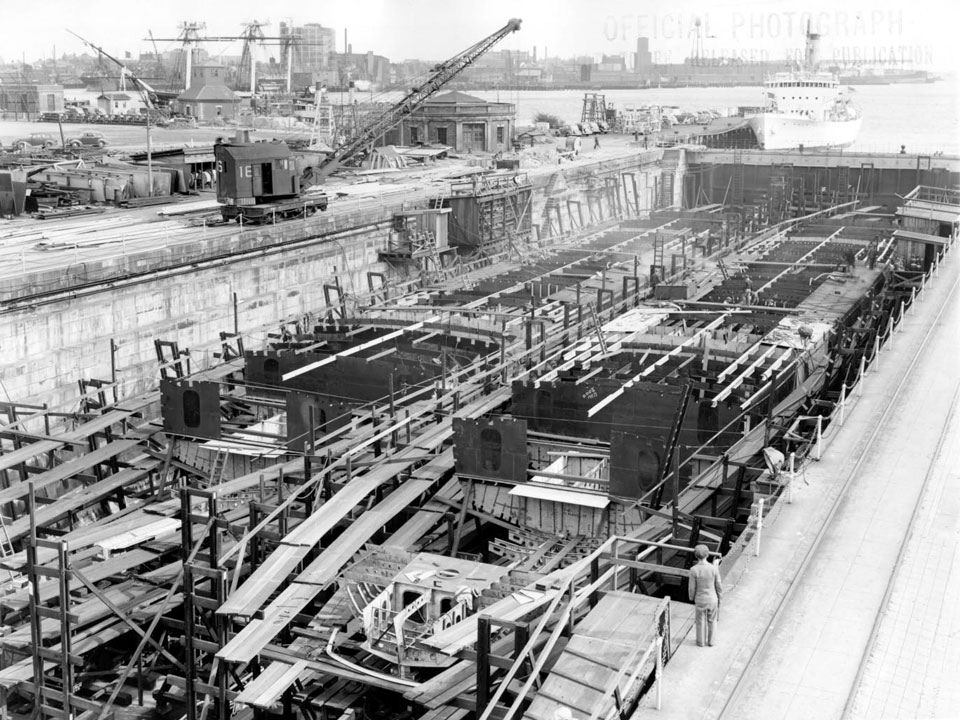The black and white photograph captures an outdoor industrial setting centered around a construction site near the ocean. A mix of wooden boards, metallic poles, and various scaffolding structures litter the scene, suggesting an ongoing shipbuilding project. Several machines, including a large vehicle with a crane, are scattered throughout the site, aiding in the construction efforts. In the midst of this industrial chaos, a young person or boy, distinguished by his short stature and wearing a hat, stands near a street and gazes out into the distance. The top right of the image offers a view of the ocean, where a large white ship is anchored, reinforcing the notion that this could be a port or shipping dock. In the distant background, additional buildings and industrial elements are faintly visible.